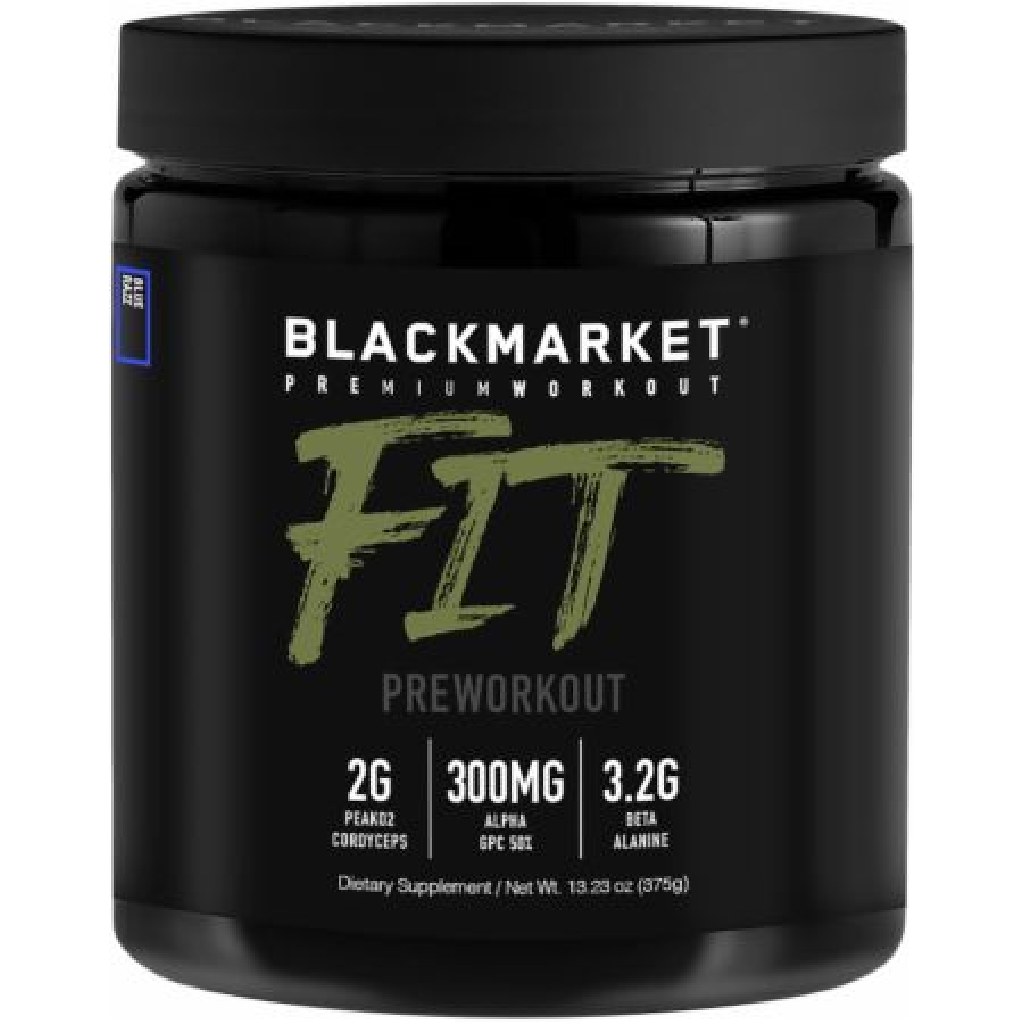This is a close-up photograph of a black, cylindrical, plastic jar with a black screw-top lid. The jar is adorned with a black label featuring an array of text. Prominently displayed at the top in white lettering is "Black Market Premium Workout." Dominating the center of the label is the word "FIT" written in large, green, brushstroke-style text. Below this, in gray, it reads "pre-workout," followed by several nutritional details: "2G Peak O2 Cordyceps," "300mg Alpha GPC-58," and "3.2g Beta-Alanine." The label also states that it is a dietary supplement and provides net weight details, marked as 13.23 ounces (375 grams). The image has a plain white background, highlighting the product as one might see on an e-retailer site.